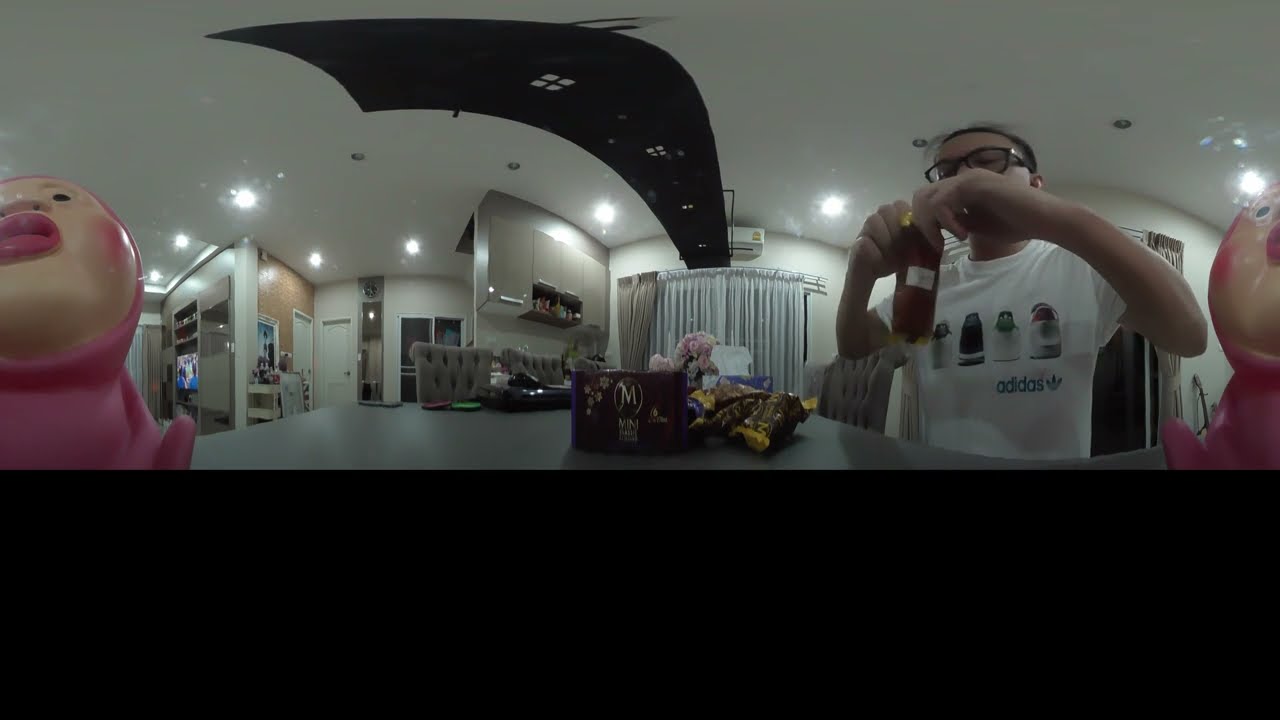In this detailed and intriguing image, we observe a man holding a tube-like object with a red and gold wrapper, suggesting it could be a type of food about to be unwrapped. He is a somewhat skinny, balding individual wearing a white t-shirt and thick black glasses, positioned in what appears to be a living room with white and beige curtains behind him. A large box, likely from which the object was extracted, sits on a gray table with gray cushioned seats around it, resembling a dining room setting. This box features an "M" and the word "Mini" on it. The background includes various pieces of furniture, some hints of a kitchen, and a statue-like object on the left side. The image's lighting and coloration are predominantly light gray with white circles dispersed throughout and a mix of colors including black, peach, pink, tan, gray, white, brown, purple, and yellow, suggesting it's nighttime indoors. The photo appears slightly warped, revealing more peculiar shapes, like a machete-like black shape above the white curtains.